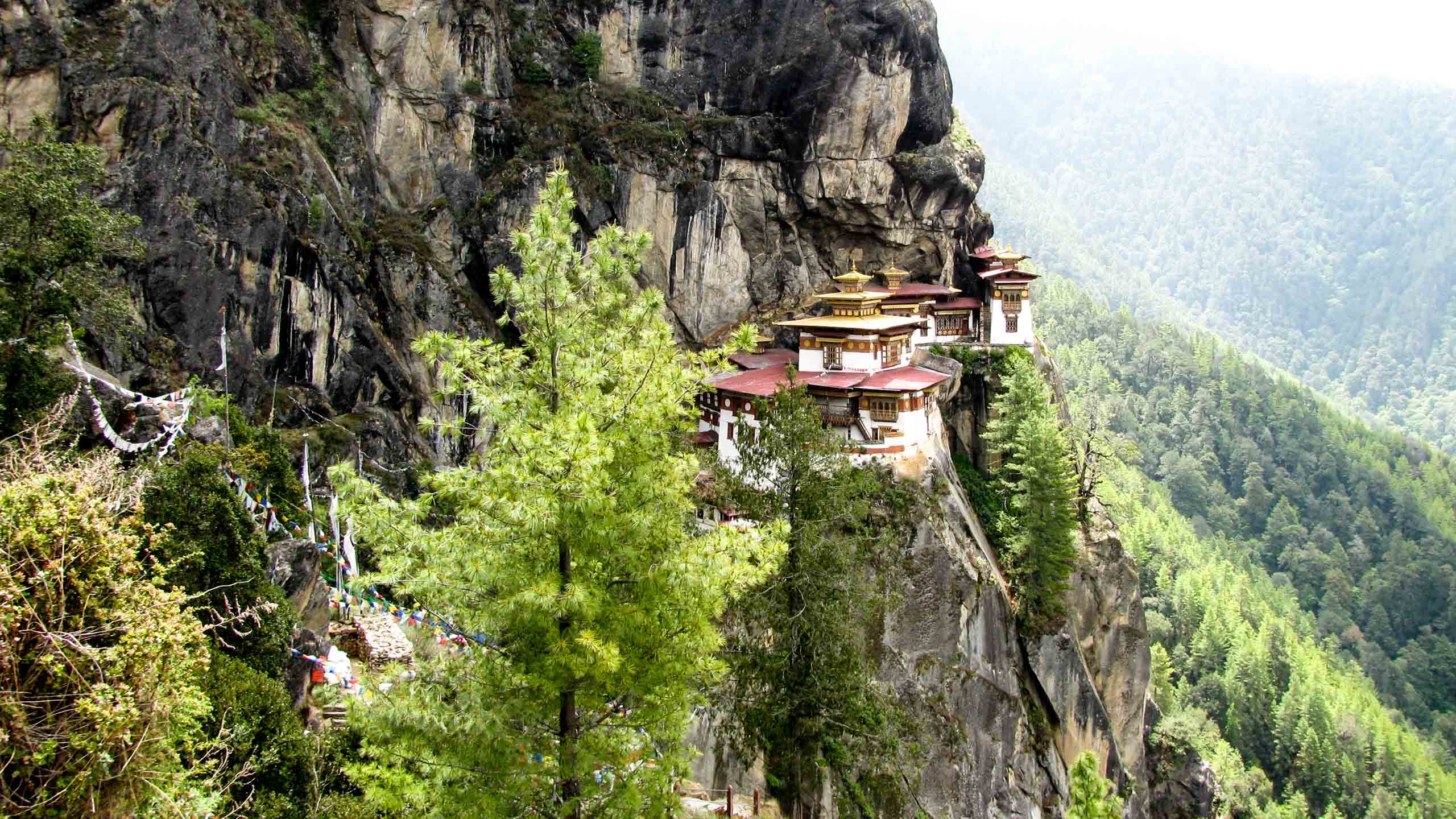This image, taken from a high vantage point, captures the dramatic and majestic Paro Taktsang Buddhist Temple in Bhutan, also known as the Hidden Kingdom. This vertically aligned photograph offers an aerial view of the temple complex, which is perched precariously on the edge of a sheer rock cliff. The central structure features a striking white facade with a red-tiled roof, and atop this sits another section with a gold roof, adorned with statues. The pagoda-like design is distinctly Asian, evoking a sense of cultural and architectural heritage.

The landscape around the temple is equally breathtaking. The left side of the image reveals the gray, rocky expanse of the cliffside, while the right side descends steeply into a forest of tall green trees. The background merges into a misty, hilly terrain, dotted with more trees and bathed in a lighter hue from the sunlight filtering through the fog. The upper right corner of the photograph includes a glimpse of the bright sky, enhancing the ethereal quality of the scene. The temple, with its multi-level roofs and intricate statues, stands as a testament to human ingenuity and spiritual devotion, blending seamlessly into the rugged yet tranquil mountainous landscape.